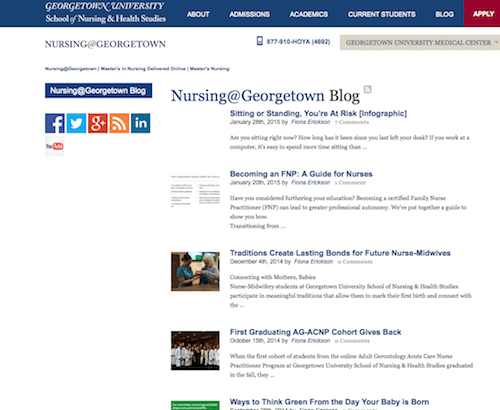A screenshot of the Georgetown University School of Nursing and Health Studies webpage is displayed. The page features a clean, primarily white background with black text, complemented by blue links. The top navigation menu is blue and includes essential links such as admissions, academics, current students, blog, and apply. On the left side of the screen, there are fewer links, including social media icons for Facebook, Twitter, Google+, LinkedIn, YouTube, and an RSS feed. An 877 contact number is also visible. The central section of the page showcases a variety of blog posts related to nursing, including topics like the risks of sitting or standing, becoming a Family Nurse Practitioner (FNP), traditions among nurse midwives, charitable efforts by the first graduating cohort, and eco-friendly practices for newborn care. The word "Hoya" can be seen, indicating the team name.